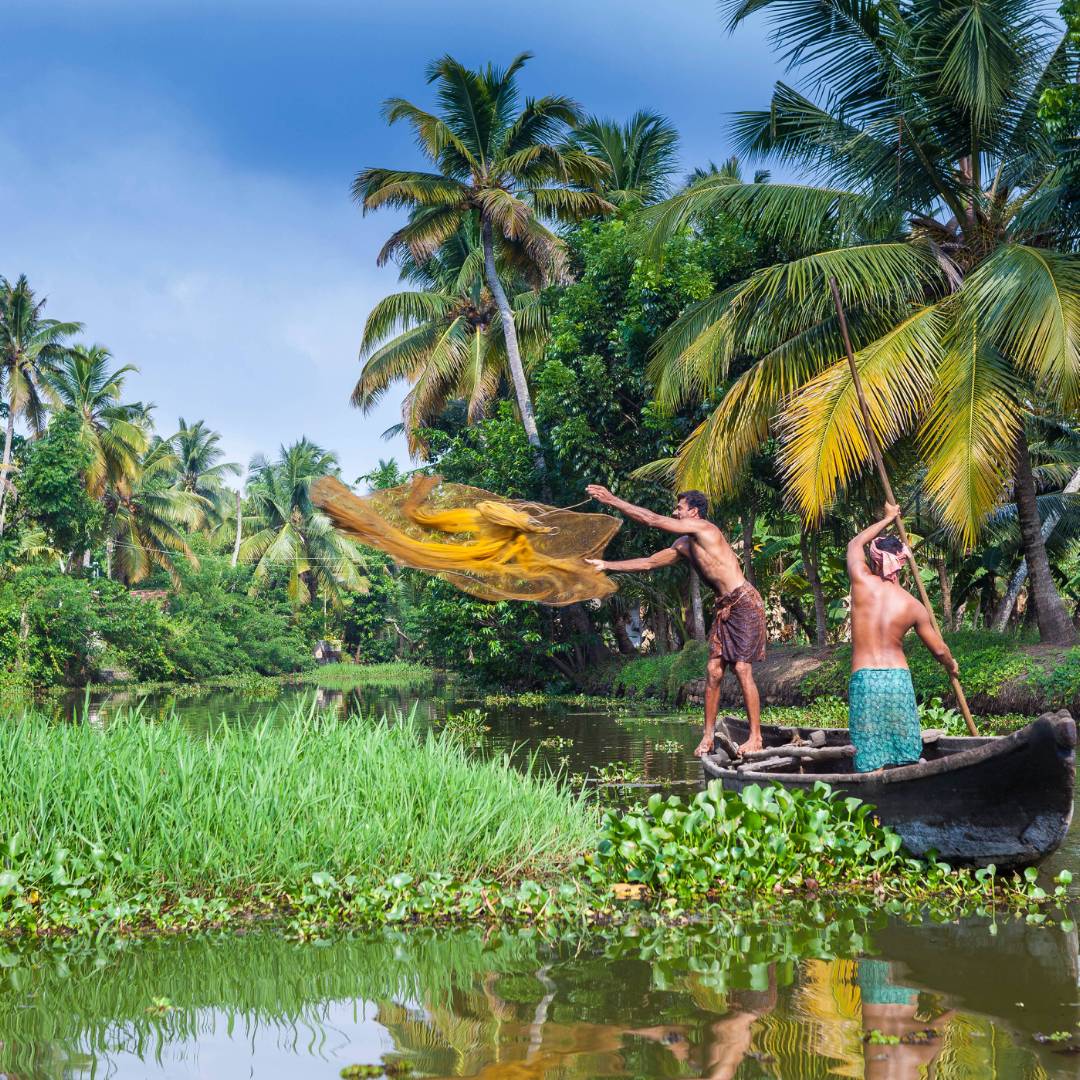In the photograph, two men are skillfully balancing in a basic canoe within a lush, tropical lagoon. The verdant backdrop is filled with palm trees, green plants, and bushes, enveloping the scene in a swampy, Costa Rica-like ambiance. The water, which appears somewhat brackish, reflects the image of the men and their boat, illustrating the tranquil yet vibrant environment. 

The man at the front edge of the canoe, dressed in wet brown shorts, is captured mid-action, precariously tossing a golden-yellow net into the water with both arms outstretched. His position at the edge of the boat and his concentration reveal a high level of expertise. The other man, standing more stably at the rear of the canoe, is wearing a blue-patterned sarong and a head wrap. He holds a long oar, twice his height, which he uses to navigate the canoe through the water, reminiscent of a gondolier. The sunlight bathes the scene, casting reflections and highlighting the clear blue sky with faint, wispy clouds, enhancing the photograph's tropical, serene beauty. The men, likely Indonesian or Indian, appear engaged in the traditional practice of fishing amidst this exotic natural setting.